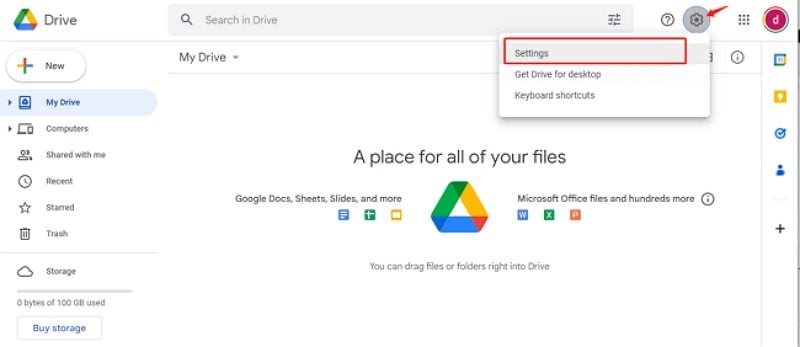The image features several elements arranged in a structured and organized layout:

1. **Top Left Corner:**
   - A multi-colored triangle composed of green, blue, and yellow segments.
   - The word "Drive" is displayed next to the triangle.

2. **Next to "Drive":**
   - A gray rectangle with a magnifying glass icon inside it.
   - The text "Search in Drive" appears within the gray rectangle.
   - On the right side of the rectangle, an unidentified symbol can be seen.
   
3. **Helpful Icons:**
   - An outlined circle with a question mark inside it.
   - A gray circle with a gear symbol, to which a red arrow points from the right.
   
4. **Settings Section:**
   - A red-outlined rectangle with the word "Settings."
   - Below this is a white rectangle containing the previous red-outlined rectangle.
   - Following this, the text "Get Drive for Desktop Keyboard Shortcuts" is displayed.

5. **Main Navigation:**
   - A square made of dots and a circle containing an indistinct letter.
   - A multi-colored plus sign next to the text "New."
   - To the right is "My Drive" with an arrow pointing downwards.
   - Below this is a gray separator line.

6. **Icons and Labels:**
   - A circle with an eye symbol.
   - A blue symbol with a small yellow detail.
   - Below these are several icons and corresponding labels: possibly "Computers," an icon representing people, a clock, a star, and a trash can – each followed by their respective labels.

7. **Additional Options:**
   - Another gray separator line followed by a cloud icon with corresponding text.
   - Another gray separator line beneath which gray text can be seen.
   - A gray-outlined rectangle with the words "Buy Storage."

8. **Main Message:**
   - A central message stating "A Place for All Your Files."
   - Some smaller black text beneath the message.
   - To the right of this, another multi-colored triangle with accompanying text.
   - Small symbols and further text that are too diminutive to discern clearly.

9. **Right-hand Sidebar:**
   - A yellow square with a dot in the center.
   - A blue, indiscernible object.
   - A blue person symbol next to a plus sign.

The layout and rich array of icons and text suggest a detailed interface, perhaps of a software or online storage service.